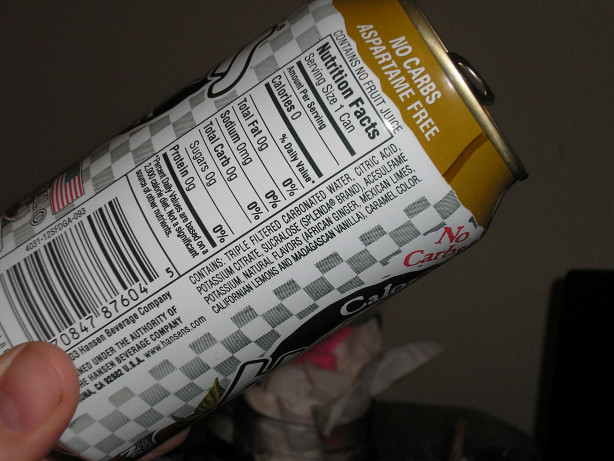The photograph showcases the back label of an aluminum can, likely a Hansen's soda, being held and tilted slightly up and to the right. The can features a white and gray checkered label with a tan-gold top section. Prominently displayed around the top lip are the phrases "no carbs" and "aspartame free." The label details the nutrition facts, revealing zero calories, fat, sodium, carbs, sugar, and protein per serving, with the serving size being one can. It also specifies that the beverage contains no fruit juice. Ingredients listed on the label include triple filtered carbonated water, citric acid, potassium citrate, sucralose (Splenda brand), acesulfame potassium, natural flavors, African ginger, Mexican limes, Californian lemons, Madagascan vanilla, and caramel color. Information about the Hansen's Beverage Company is visible, though a finger partially obscures the first digits of the UPC code. An American flag is also present on the label.